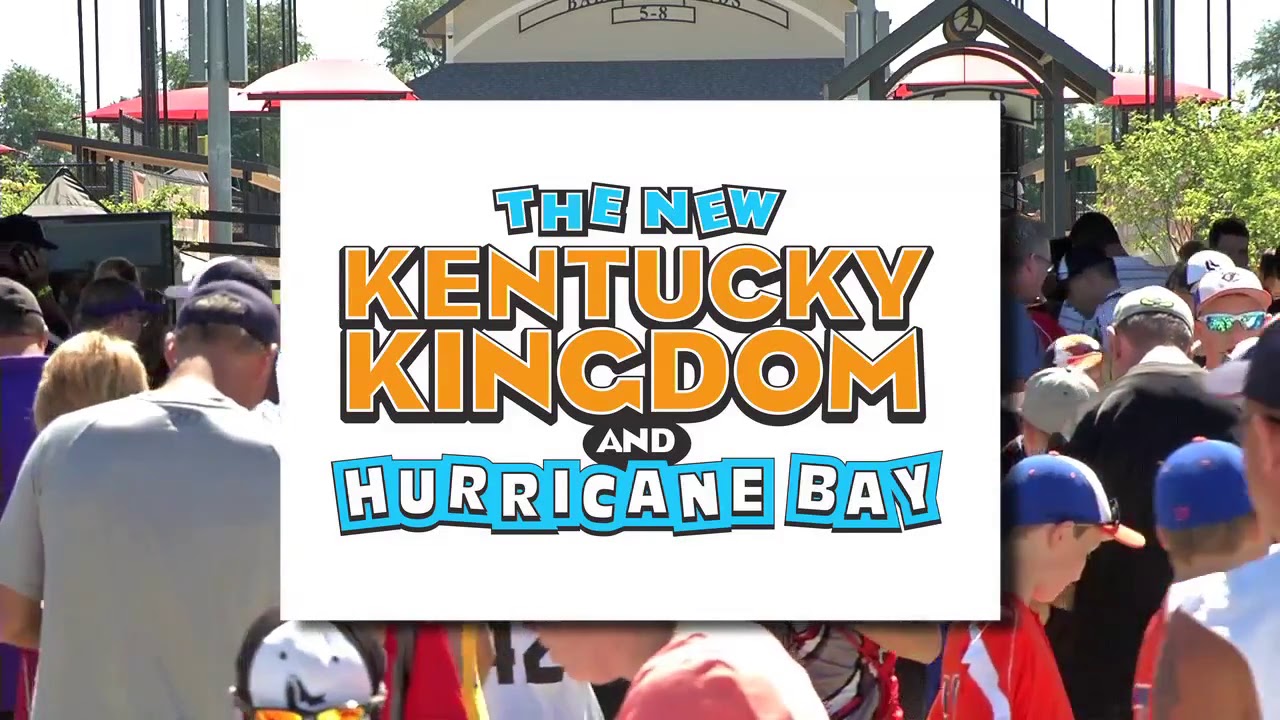The image prominently features a lively, outdoor scene at what appears to be an amusement park, where a large crowd of people, most of them wearing baseball caps in various colors, are gathered. The crowd is diverse, including both adults, likely in their 30s and 40s, and children around 10 years old. Most are dressed in light, summer or spring clothing, suggesting a warm day. They seem to be milling around or perhaps waiting in line to enter an attraction.

At the center of the image is a large white box, serving as a sign. In bold, light blue all-caps letters, it reads "THE NEW," followed by "KENTUCKY" in orange and "KINGDOM" in a similar orange beneath it. Below this, within a little black circle with white lettering, it says "AND." Adjacent to this, in white letters outlined in the same light blue, it says "HURRICANE BAY." The background of the sign is white, contrasting with the colorful lettering. Surrounding this central sign, the photograph captures the bustling atmosphere of the parkgoers, who are positioned against a backdrop of green bushes and various poles, enhancing the energetic and vibrant feel of the scene.